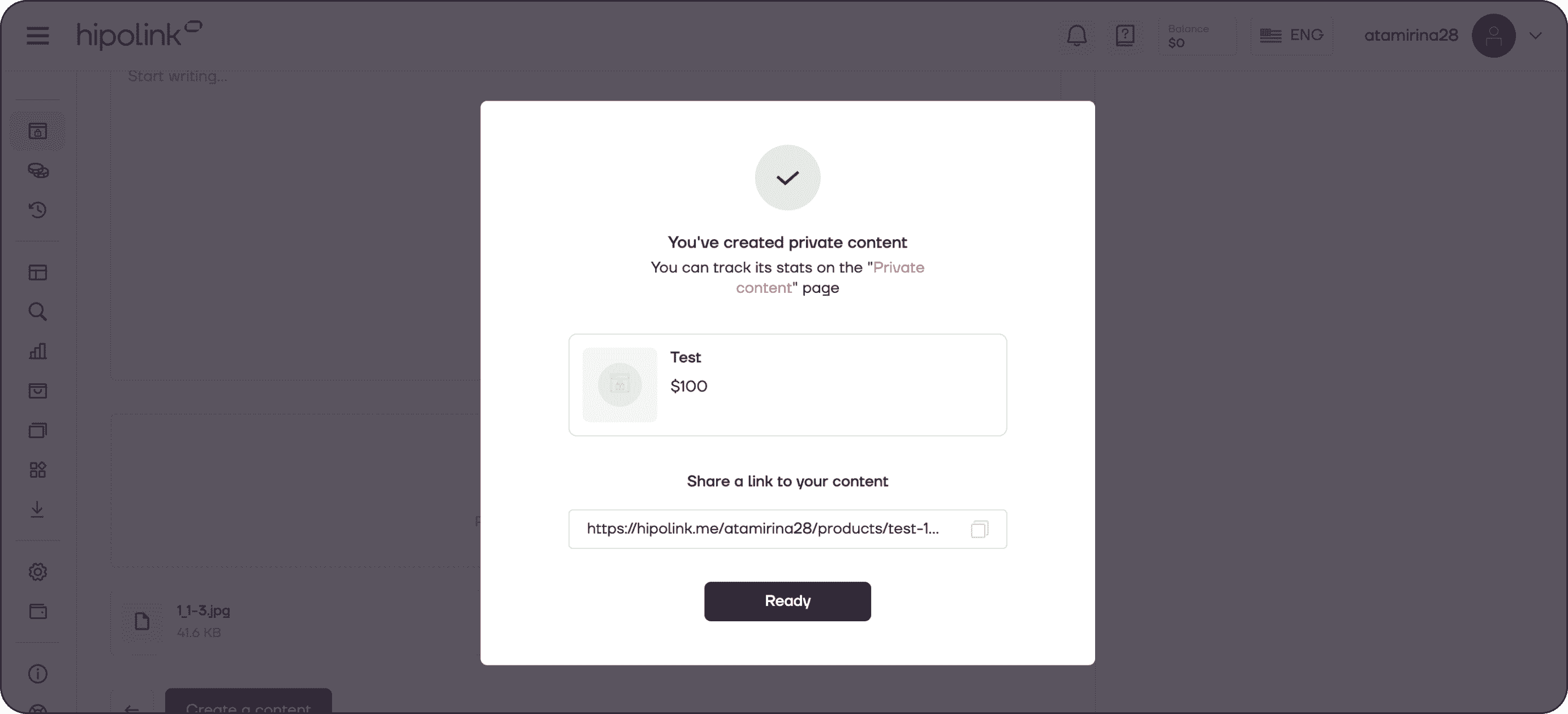The image portrays a webpage from a site named "Hypolink," as indicated by the logo on the top-left corner. On the left side of the page, a vertical taskbar features a hamburger menu at the top, followed by various icons representing different sections of the site, such as a car, a magnifying glass, a bar chart, file boxes, and a settings gear.

In the upper right section, the user's information is displayed. The username "Atamirina28" accompanies a generic profile icon illustrating a person. Further right, the user's language setting is shown as English, alongside their balance, which is currently zero dollars. Adjacent to these details are icons for notifications and help: a notification bell and a question mark, respectively.

Centrally located is a pop-up notification against a white background with predominantly black text, accented by red text for emphasis. It reads: "You've created private content," emphasizing "private content" in red. It further informs the user that they can track stats on the private content page. The private content is titled "Test" and has an associated value of $100. It includes a shareable link and a prominent black button labeled "Ready" in white.

Behind the pop-up, a JPG file named "113.jpg" is visible, with a size of 41.6 kilobytes. Below this file, there is a button labeled "Create Content," suggesting further user interaction options.